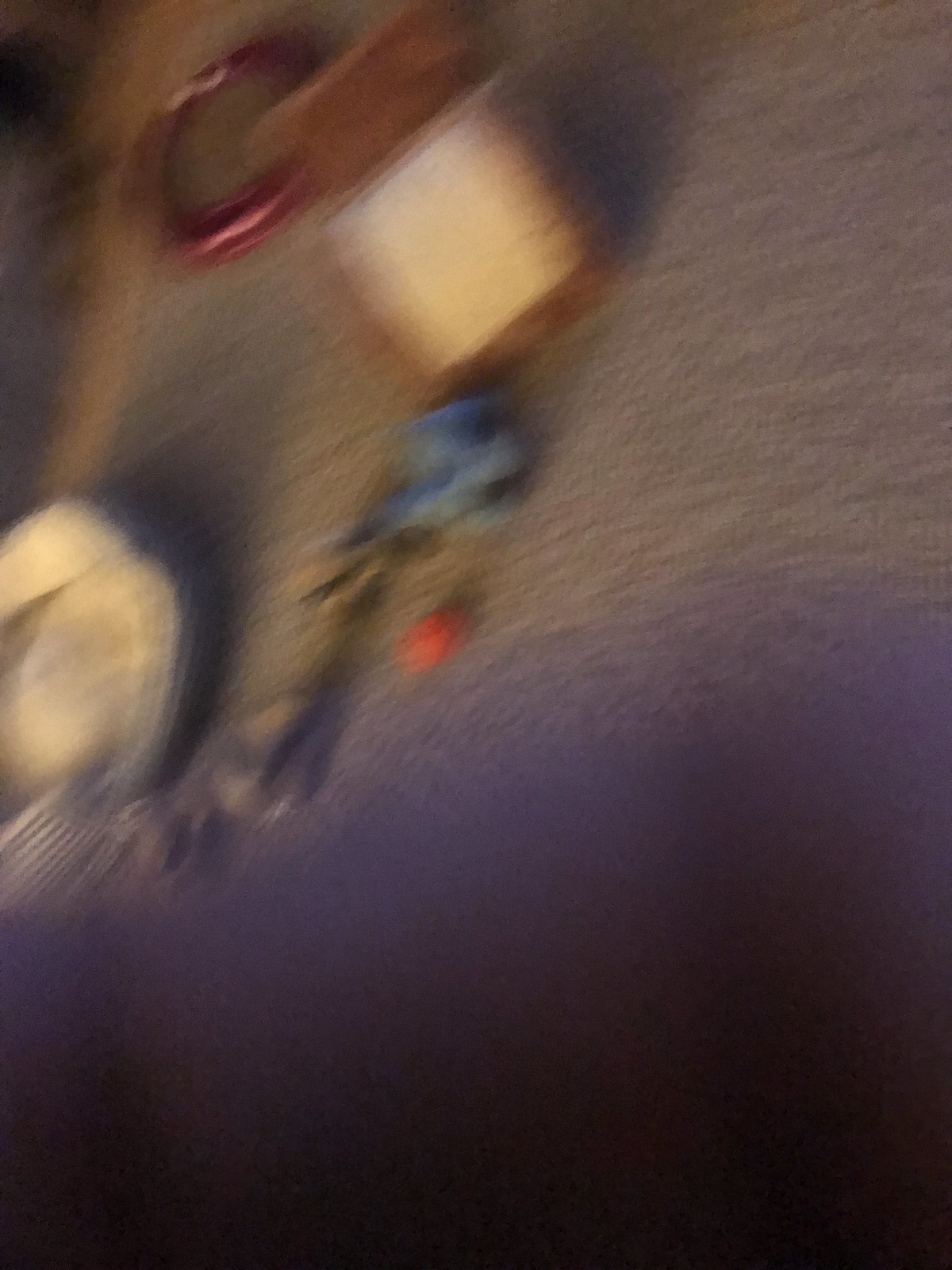This image captures a somewhat chaotic and blurry scene of various dog toys scattered across a gray rug on the floor. The photograph, seemingly taken accidentally at an odd angle, likely when someone was rising from a seated position, features an assortment of playthings: a red ball, a long rope toy, and a small dog bed. Additionally, there is a scratching post, brown with a white front, adding to the perplexing array. The top right corner of the image reveals a glimpse of a tan-colored floor, possibly wood or tile, although the overall focus remains elusive, casting everything in a hazy blur.